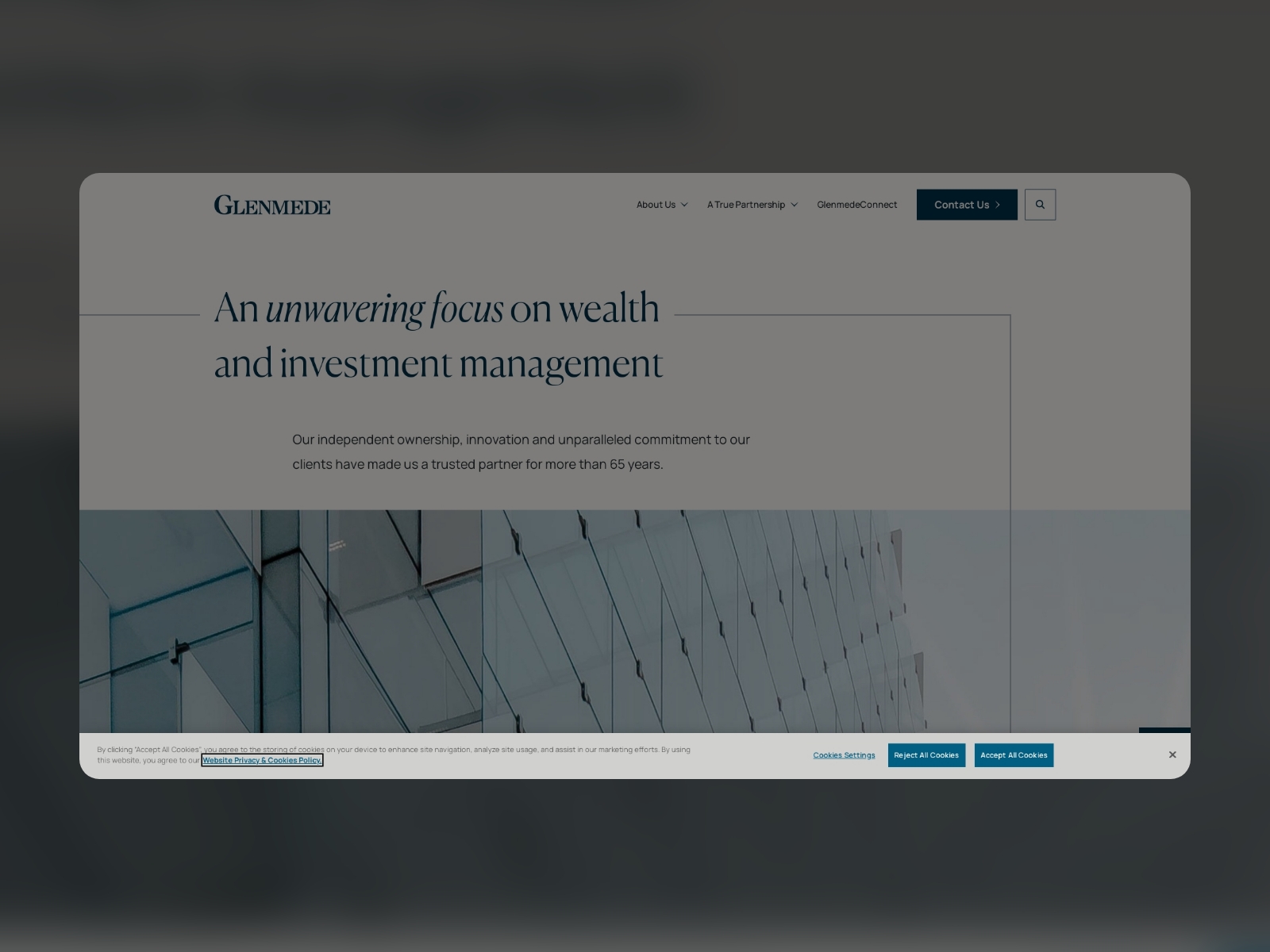The image predominantly features a grayscale theme. Against a dark gray background that borders on black, there is a central light gray rectangle occupying the upper half of the image. At the very top of this rectangle is the name "Glenn Meade" in bold, uppercase letters. To the right of this title, the words "About Us" are followed by a downward arrow, and next to it, "A True Partnership" is also followed by a downward arrow. Further along, the text reads "Something Connect" and "Contact Us" which are set against a black background, accompanied by a white rectangle with a magnifying glass icon.

Below this header, the phrase "We have an unwavering focus on wealth" is prominently displayed, with "unwavering focus" in italics for emphasis. Beneath this headline, the phrase "And Investment Management" appears, followed by a description in smaller print: "Our Independent Ownership, Innovation, and Unparalleled Commitment to our Clients have made us a trusted partner for more than 65 years."

Additionally, there is an abstract image composed of geometric shapes in shades of grayish blue. At the very bottom, there is another line of text, but it is too small to be legible.